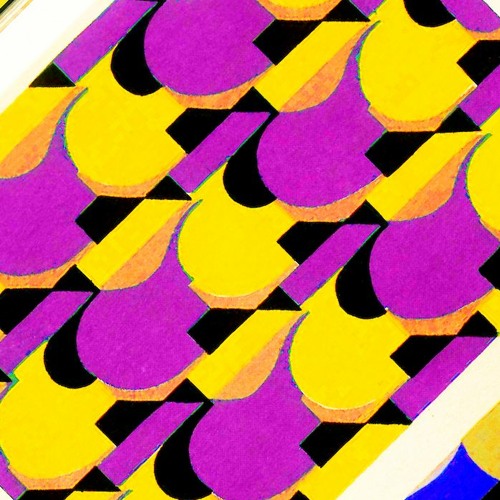This abstract painting is a vibrant and intricate composition featuring a blend of purple, black, and yellow hues. The painting is square-shaped, with a base layer of darker mustard yellow. It showcases a series of about four parallel diagonal lines, running across the canvas and consisting of a mix of purple, black, and yellow. Between these diagonal lines, the space is filled with more rounded and organic shapes, predominantly circles and bean-like forms, also in purple, black, and yellow. These alternating and overlapping shapes create a dynamic and funky geometric pattern that draws the eye and evokes a sense of abstract, modern artistry.